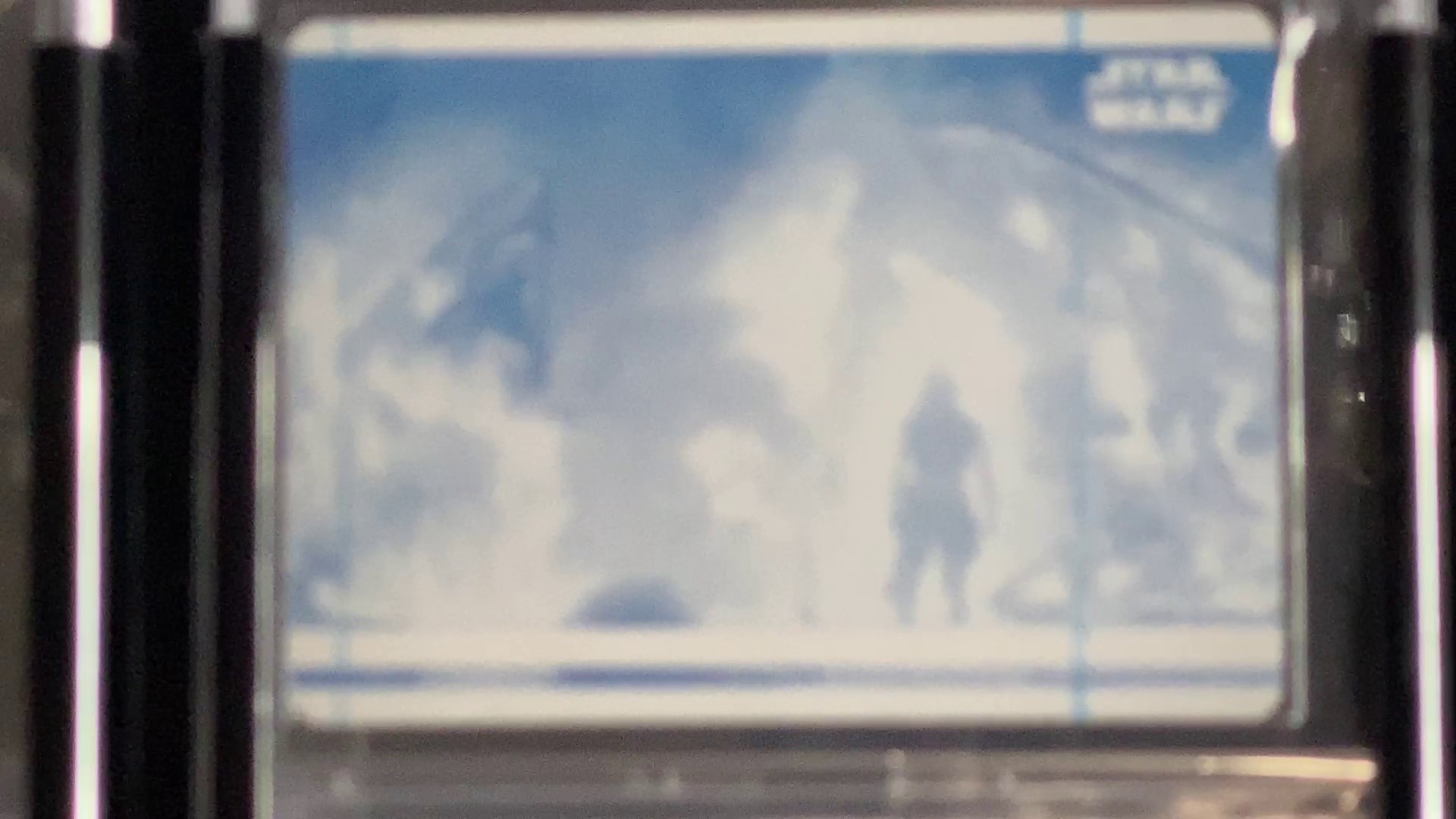This image showcases a slightly blurry photograph, seemingly of a picture or trading card. At the top corner, the unmistakable trademark lettering of "Star Wars" is prominently displayed, indicating its association with the iconic franchise. The visual composition appears to include a silhouette of a character standing on a glacial, icy planet dominated by various shades of blue and white, suggesting it could be the planet Hoth. Flanking either side of the image, there are indistinct black cylindrical objects that might be part of a decorative frame or surrounding elements within the scene.